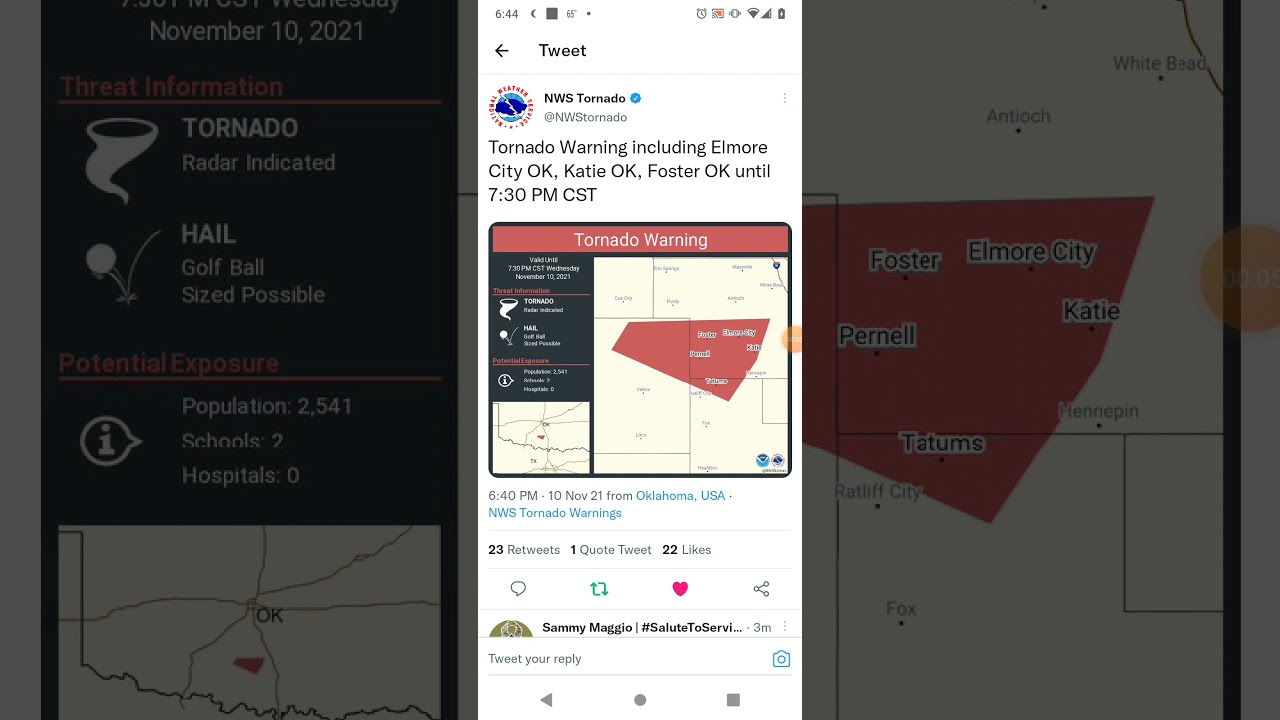Detailing both the main central content and the background overlaid area vividly:

The image captures a striking screenshot of a cell phone display, centered against a larger, dimmed background screen. Dominating the view is the vertical white phone screen, proclaiming urgent weather information. At the top of this screen, the word "Tweet" sits prominently. Below it, the Twitter handle "@NWSTornado," accompanied by a small cloud and sky icon, disseminates critical information.

The key alert reads: "Tornado Warning including Elmore City, Oklahoma, Katy, Oklahoma, Foster, Oklahoma until 7:30 p.m. CST." Just beneath this alert, a small embedded screen reiterates the warning, depicting a detailed map that highlights in red the regions at risk. This smaller visual mirrors the layout of the larger, obscured background.

Further down the phone screen, crucial details are timestamped and attributed with "Oklahoma, USA - NWS Tornado Warnings", emphasized in clickable blue text. The post has garnered engagement, noted by "23 retweets, 1 quote tweet, and 22 likes."

Shifting to the grayed-out background, the left vertical bar commands focus with the header "Threat Information" in bold red. The subsequent details read: "Tornado radar indicated," tagged with a white tornado icon, and "Hail golf ball size possible," denoted by a white circle. The section marked "Potential Exposure" follows in red, listing "Population: 2005, Schools: 2, Hospitals: 0."

Central to this background is a detailed map pinpointing Oklahoma, dramatically highlighting the tornado's anticipated impact zone in vivid red. This map zooms into Foster, Elmore City, Katy, Purnell, and Tatum's, providing a stark visual representation of the areas under threat.

In juxtaposition, the central phone screen and the encompassing background converge into a cohesive alert system, emphasizing the urgency and thoroughness of the tornado warning issued by the National Weather Service.